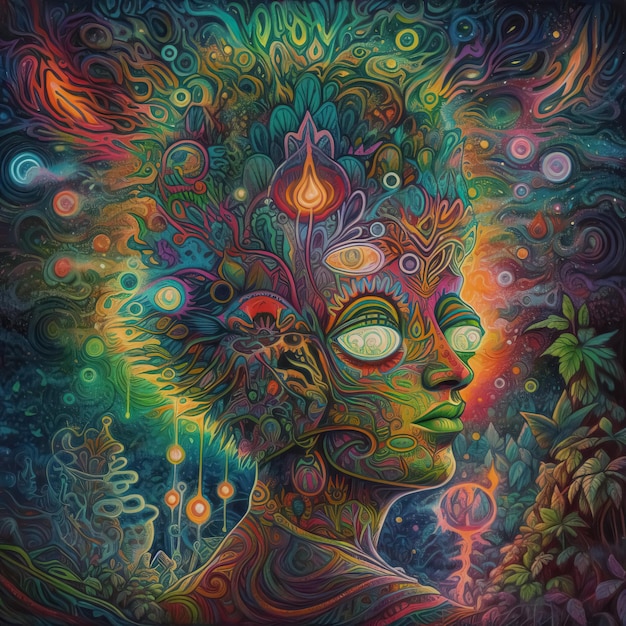The artwork is a vivid and intricate psychedelic-style painting or drawing of a woman’s head, portrayed with striking, neon-like colors against a navy blue and dark turquoise background. The right side of her face is depicted with bright, pale green eyes detailed with swirling patterns and matching green lips. Her nose and lips are drawn with precision, while her skin and neck exhibit a mesmerizing array of swirly, tattoo-like patterns in pink, blue, and orange hues. 

Her elaborate hair resembles an afro with flamboyant spikes and curls, featuring multi-colored designs in blues, yellows, pinks, and greens. The edges of her hair are highlighted with lighter shades to create a flame-like effect, further accentuated by fire-like colors such as reds and oranges emanating from the top. Additionally, some sections of her hair are detailed with teardrop shapes and peacock feather-like designs, adding to the cosmic and surreal vibe.

Surrounding the woman are numerous intricate and swirling designs, including alien-like plant features, vibrant leaves, bushes, and vines in myriad colors such as greens, blues, and purples. These botanical elements are dispersed around her, contributing to the overall dynamic and mesmerizing composition of the artwork.